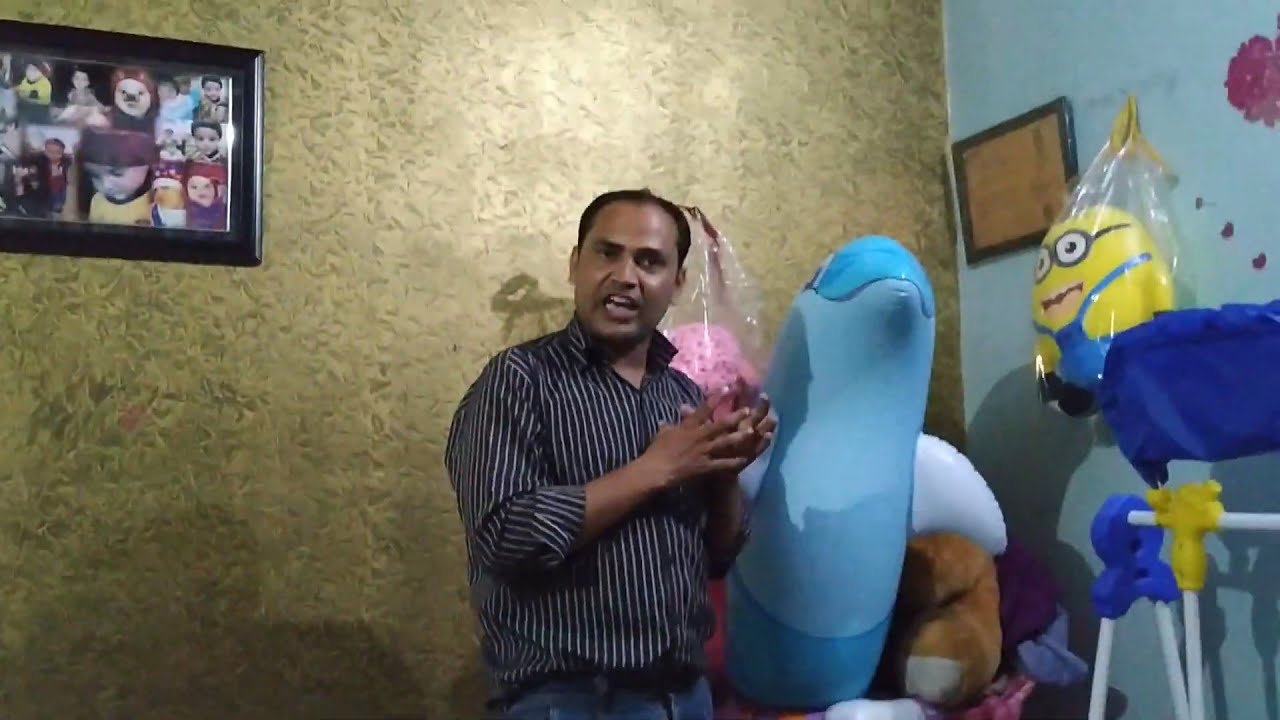A horizontal rectangular photograph captures a man standing in the corner of a child's playroom, surrounded by an assortment of toys. The background features a gold patterned wall transitioning into a blue wall on the right. Hanging on the gold wall in the upper left corner is a black picture frame displaying a montage of baby photographs. On the blue wall, another frame can be seen, containing an indistinguishable brown paper, and a plush Minion from *Despicable Me* wrapped in a plastic bag hangs from a hook. The man, in his thirties, has short black hair, slightly dark skin, and wears a black and white striped button-down shirt with the sleeves rolled up, paired with blue jeans. His mouth is open, his hands are held in front of him, indicating he is talking. To his right is a large blue inflatable toy, resembling a dolphin, with its head and mouth visibly protruding. The lower right corner showcases various children's toys, including blue and yellow items connected to white poles. The scene is completed by pink flowers on the wall, suggesting a vibrant and playful environment, likely a child's playroom.